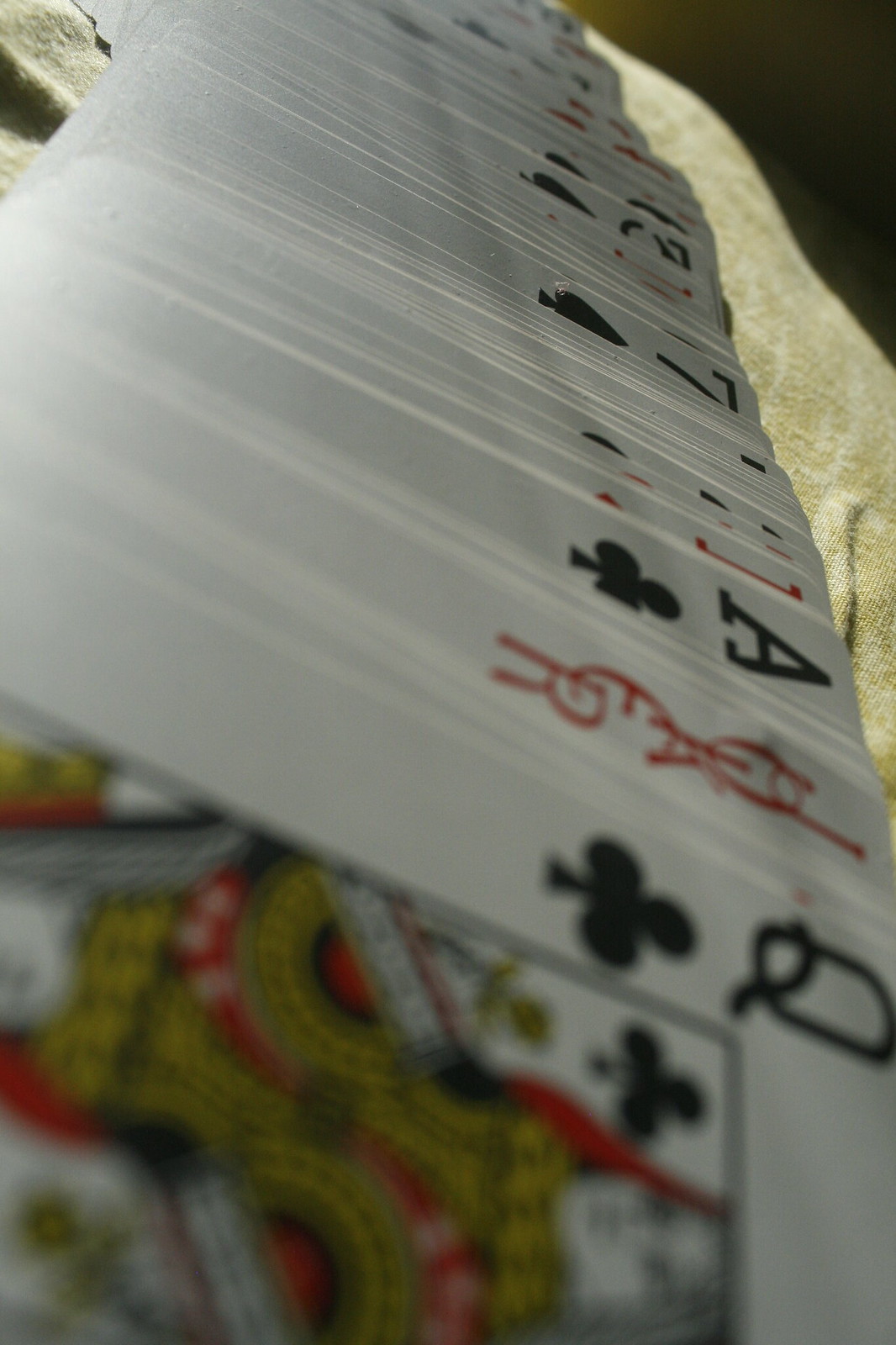A close-up photograph of a deck of cards meticulously spread in a narrow, even fan across a linen tablecloth. The tablecloth features a delicate brocade pattern with a greenish tinge on a creamy white background. The viewer's perspective is from the side, as if seated to the right of the person who arranged the cards. The top card in the spread is the Queen of Clubs, while other visible cards include a Joker adorned with ornate script (tilted so the word reads from right to left), an Ace of Clubs, a Seven of Spades, and a partially obscured Three of Spades. The foreground card is heavily blurred, drawing focus to the middle section of the spread. The background of the image fades into darkness in the upper right corner, further emphasizing the elegant display of the cards on the textured tablecloth.